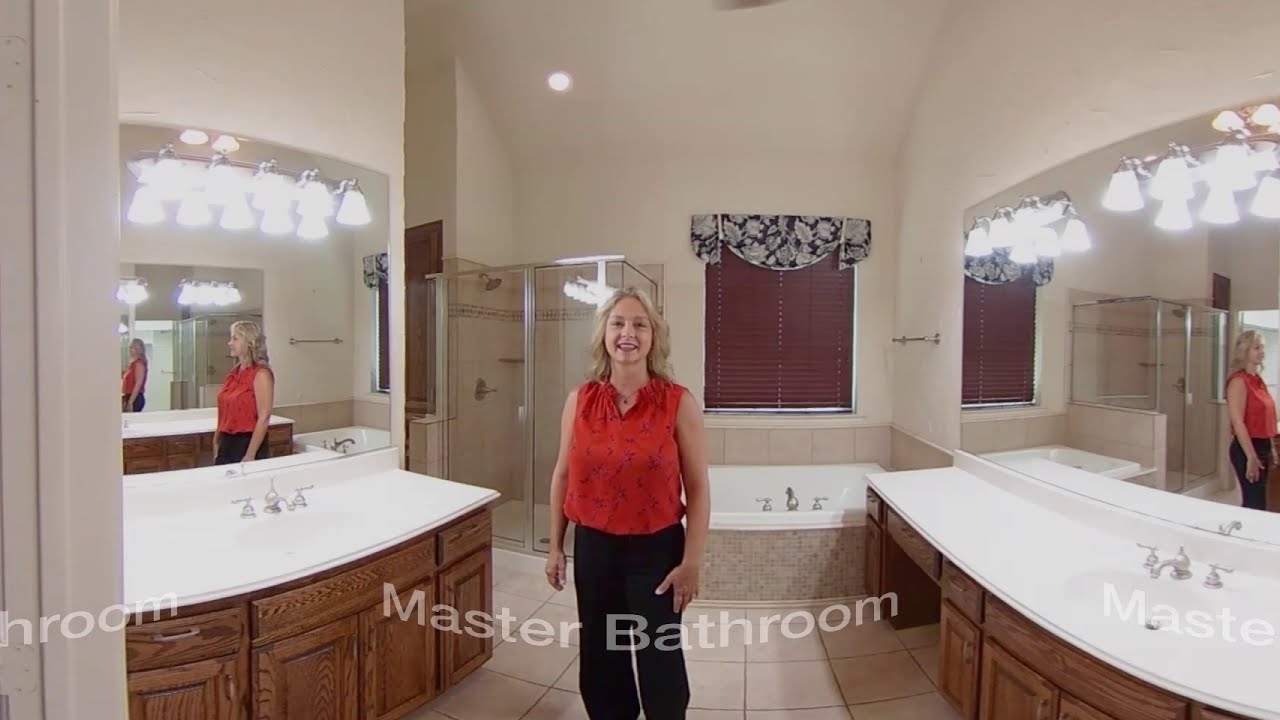The image captures a spacious and pristine master bathroom, as indicated by white letters at the bottom of the picture. The bathroom features dual sinks with white countertops and wooden cabinets beneath, positioned symmetrically on both sides. Mirrors mounted above the sinks reflect the central figure—a smiling woman with shoulder-length, blonde feathered hair. She wears a sleeveless reddish blouse with purple designs and blue jeans, though the image quality makes the exact details of her attire somewhat unclear. She also has a necklace. The bathroom's backdrop includes a visible bathtub, a window with drawn shades and a small curtain, and a transparent glass (or plastic) shower stall to the left behind her. The walls and floor of the bathroom are beige, contributing to the overall posh and high-end appearance, emphasized further by the individual light fixtures hanging on either side of the mirrors. The woman's proud and determined expression suggests she might be the homeowner or a realtor, possibly showcasing the property for sale.